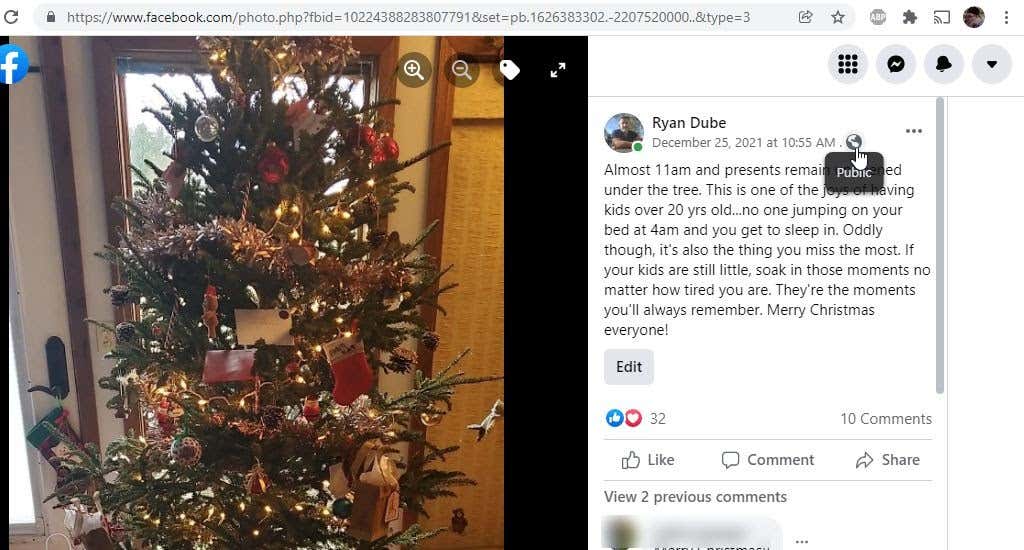**Descriptive Caption:**

In this Facebook post by Ryan Duby, dated December 25th, 2021, at 10:55 a.m., a festive Christmas scene is shared. The top of the post displays "facebook.com/photo" in the gray header, and to the right side, there's a dark, indistinguishable profile image, along with three vertical circles. Below these are additional gray circles containing other images.

The main picture showcases Ryan's Christmas tree positioned beside a glass door, which upon closer inspection, is actually a window next to the door. The tree, adorned with large ornaments relative to its size, appears rather sparse, allowing visibility through its branches. Old-fashioned garland tastefully decorates the tree, and a sizable stocking bearing Ryan's name hangs prominently.

The accompanying text in the post reads: "Almost 11 a.m. and presents remain. This is one of the joys of having kids over 20 years old. No one jumping on your bed at 4 a.m. and you get to sleep in. Oddly though, it’s also the thing you miss the most. If your kids are still little, soak in those moments no matter how tired you are. They’re the moments you'll always remember. Merry Christmas everyone."

At the bottom of the post, there is an "Edit" button, as well as options to like, comment, or share the post. It has received 32 likes and 10 comments, although the first two comments are whited out.